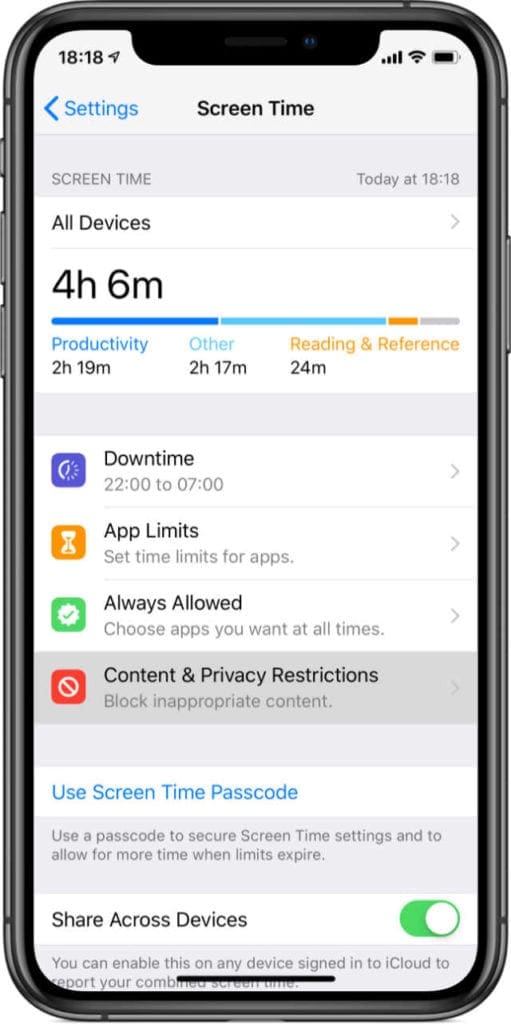The image depicts an iPhone displaying the "Screen Time" settings under the "Settings" menu. The iPhone shows a full battery icon and four bars of cellular connection, indicating strong signal strength. The time displayed on the iPhone is 18:18. At the top of the screen, the word "Settings" is highlighted in blue with a left-pointing arrow beside it.

In the center, the title "Screen Time" is prominently displayed in black text. Below it, the current screen time usage for "Today at 18:18" is given, showing a total of "4 hours 6 minutes." Categories of usage are listed beneath, with "Productivity" highlighted in blue showing "2 hours 19 minutes," "Other" also in blue with "2 hours 17 minutes," and "Reading and Reference" in gold showing "24 minutes."

A light gray bar separates these statistics from the subsequent settings. Underneath, the following options are available:

- "Downtime" from 22:00 to 07:00.
- "App Limits" for setting time constraints on apps.
- "Always Allowed," which lets the user choose apps to be accessible at all times.
- "Content and Privacy Restrictions" for blocking inappropriate content.

These options are also separated by a light gray bar. Below the bar, "Use Screen Time Passcode" is displayed in blue on a white bar. Additionally, a message in a gray bar advises, "Use a passcode to secure screen time settings and to allow for more time when limits expire."

At the very bottom, the "Share Across Devices" option is toggled on, indicated by a green switch. The description reads, "You can enable this on any device signed into iCloud to report your combined screen time."

The bottom of the phone screen is marked by a black navigation bar, completing the display.